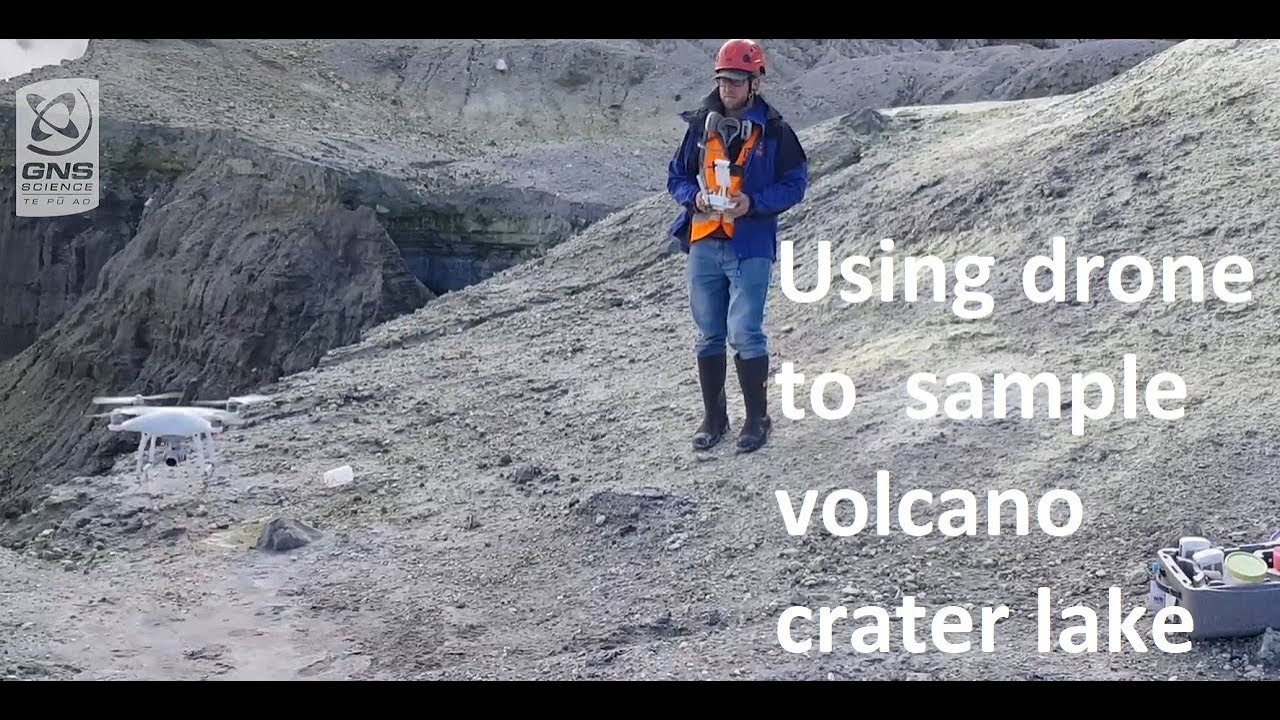A detailed photograph captured in a landscape layout, defined by black rectangular bars running along the top and bottom edges. Located in the middle of the image, a Caucasian man stands facing the camera amid a rugged, rocky, mountainous terrain. He sports blue jeans, knee-high black boots, and a layered ensemble consisting of a blue and black jacket topped with an orange safety vest. His headgear consists of a red helmet over a billed hat, and he wears glasses, potentially accompanied by facial hair. The man holds a white controller for a drone in his hands. 

In the lower left corner, a white drone equipped with a black camera is visible, ready for operation. The upper left corner features a logo with an atomic design and the text "GNS Science," possibly indicative of an organization related to geological or volcanic study. To the right of the man, text reads "using drone to sample volcano crater lake," clearly indicating an ongoing scientific endeavor. Another notable detail is a gray box situated in the bottom right corner, containing assorted items including a green lid, two clear bottles with white lids, and a red object, suggestive of field equipment or a lunchbox. The image's precise composition and contextual elements effectively convey a scene of geological exploration and drone usage amidst a volcanic landscape.